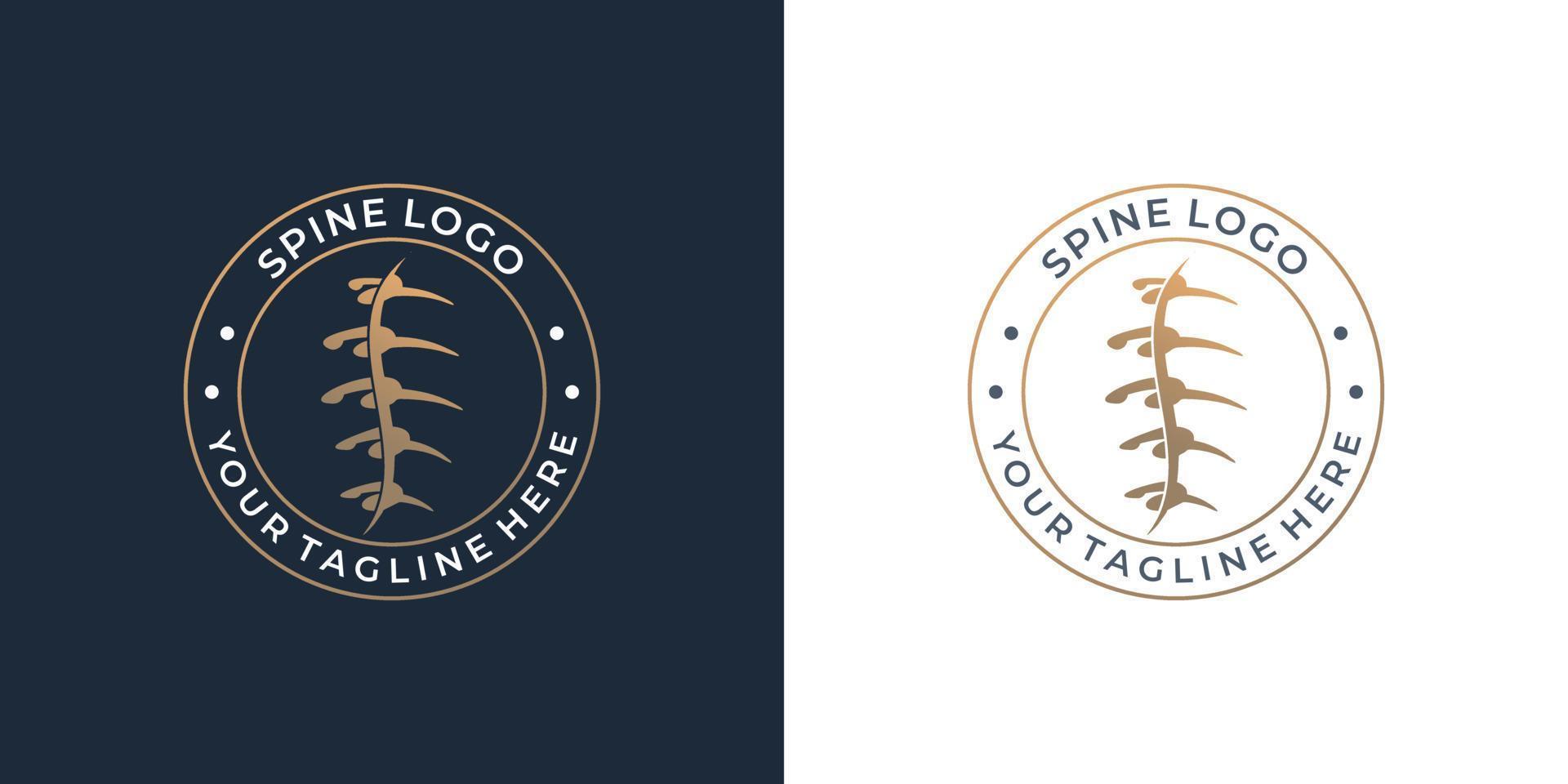The image features two side-by-side logo illustrations showcasing a staff name “Spine Logo” at the top and “Your Tagline Here” at the bottom, both encapsulated within circular designs. The left logo is set against a dark background that combines shades of blue and black, featuring gold thin-line circles and white uppercase text. An illustration of a human spine in yellow-gold occupies the central space. Conversely, the right logo mirrors this design but with a white background, black text, and the same golden spine illustration.